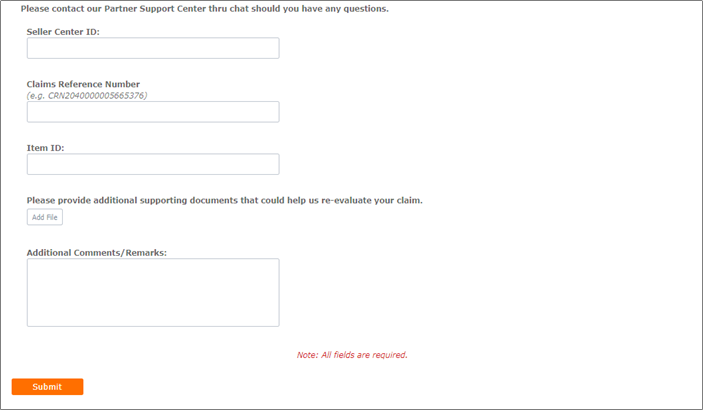The image shows a user interface form designed for individuals to fill out. The form is predominantly white with various sections outlined in gray. At the top, there is a directive stating, "Please contact our partner support center through chat should you have any questions." 

Below this, there are fields labeled "Seller's Center ID" and "Claims Reference Number," the latter of which includes an example format indicating that the first three characters should be letters followed by numbers. Another field titled "Item ID" is also present, each of these fields encased in grey outlines similar to the others.

Further down, the form requests, "Please provide additional supporting documents that could help us re-evaluate your claim," accompanied by a small button labeled "Add File" for uploading these documents. 

Next, there is a section titled "Additional Comments/Remarks" with a text box where users can type in their information. 

In small red print, the form notes that "All fields are required." At the bottom of the form, an orange "Submit" button is available for submission of the provided information.